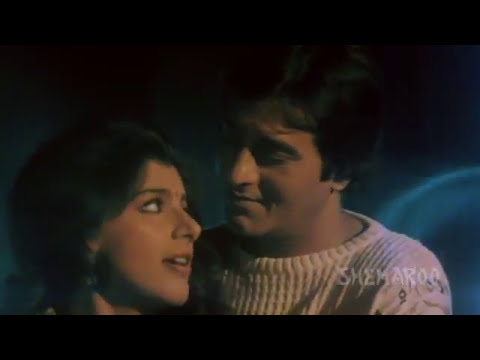The image features an Asian couple set against a dark, possibly black, background with a faint blue light illuminating their surroundings. On the left side of the image is a young woman with fluffy black or dark brown hair, adorned with a red dot between her eyebrows, which suggests cultural significance. She has brown skin, black eyebrows, and her mouth is slightly open, revealing her top teeth. Her head is turned slightly towards the man on her right, her eyes looking up at him. The man, positioned on the right, has short dark brown hair and a more mature appearance. He is wearing a white, threaded crewneck sweater and has a slight, closed-mouth smile. The man’s eyes are closed as he looks down at the woman below him. In the bottom right corner of the image, there is a semi-transparent logo in all capital letters that reads "SHIMAROO." The couple is in close proximity, appearing to share a subtle, yet intimate moment.